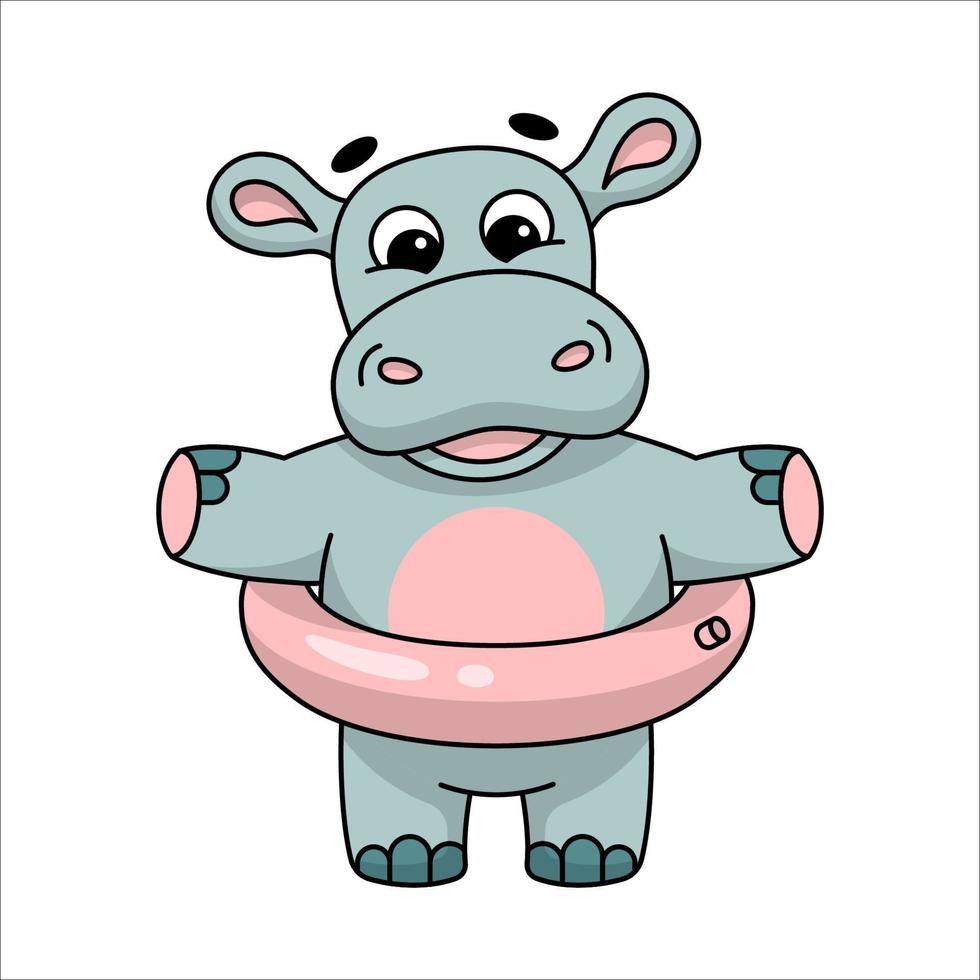The image depicts a colorful animated hippo standing upright on a white background. The hippo is primarily a grayish-blue color with pink details such as the interior of its ears, nostrils, mouth, the bottom of its paws, and its belly. It has darker blue nails on both its hands and feet. The hippo's arms are extended sideways, and around its waist is a pink inner tube with the inflatable portion clearly visible on the right side. The hippo is smiling with its mouth open and has wide, expressive eyes, accented by eyebrows perched high above its head. The overall appearance is lively and cheerful, with a playful pose suggesting it's ready for a swim.